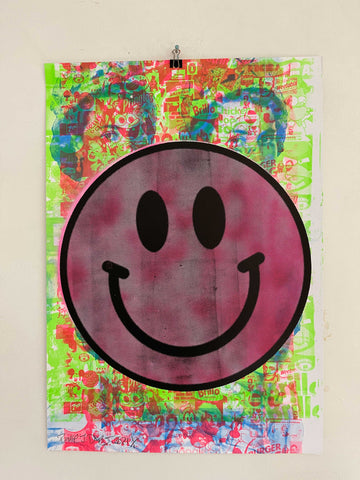This vividly detailed artwork, reminiscent of pop art, prominently features a large, circular happy face at its center. The happy face is characterized by its maroon and dark pink hues interspersed with patches of white and cream. Its striking black eyes and wide, cheerful smile contrast sharply against the vibrant colors surrounding it. The backdrop of the piece showcases a psychedelic blend of randomly applied brushstrokes in bright blue, yellow, red, green, and pink. Intriguingly, two blue, 1940s-style characters flank the smiley face, adding a whimsical touch. The collage effect is further enhanced by numerous hot pink stickers, portraying various brand images and pop culture icons such as Spongebob. The entire artwork, which is approximately the size of a large stamp or a 50-cent piece and a half, is mounted on a tan or beige background and pinned at the top with a black pin. The detailing extends to intricate, artistically rendered images of Queen Elizabeth, placed subtly in the backdrop, providing a historical juxtaposition against the modern, playful aesthetics of the piece.